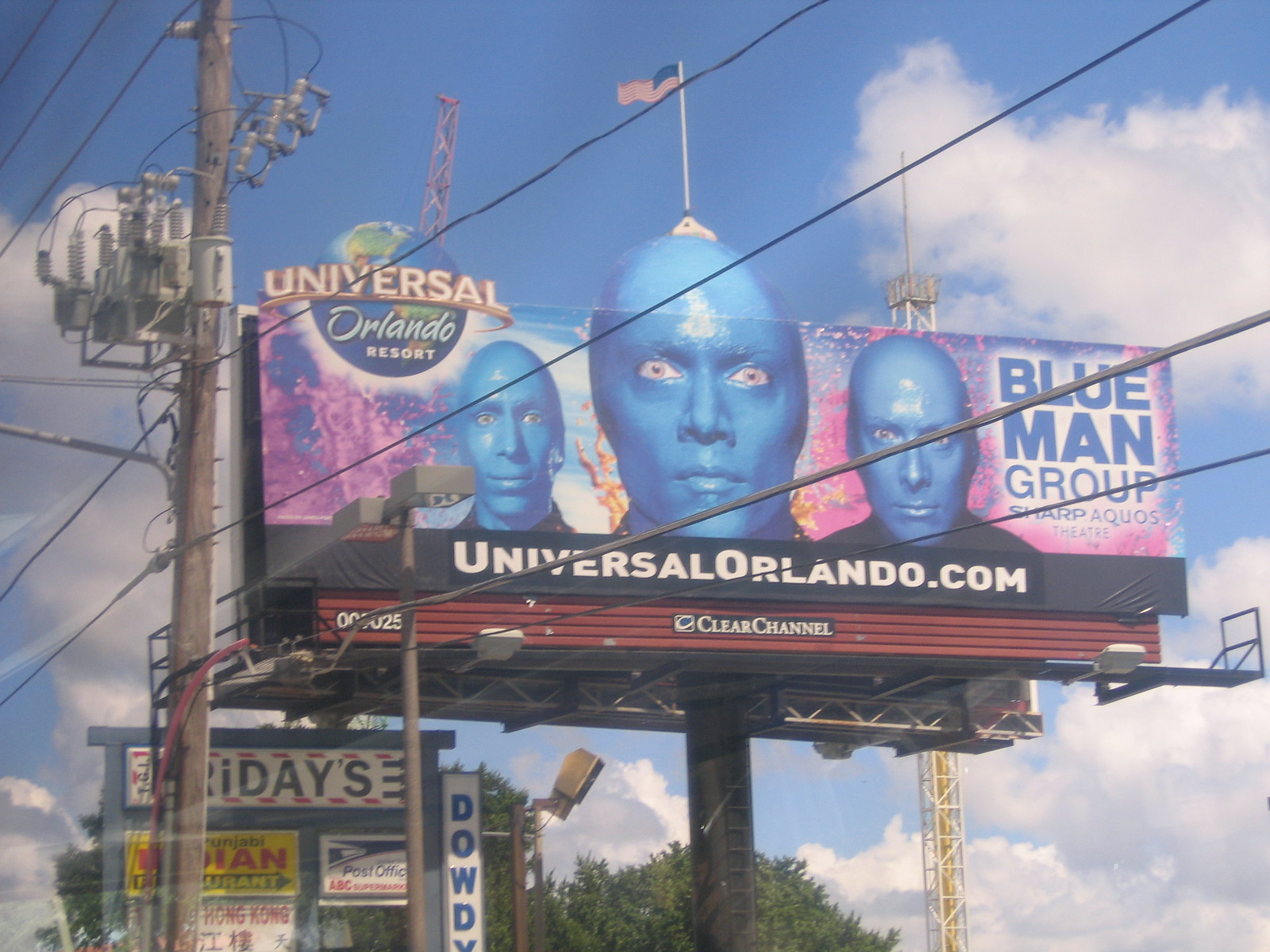This photograph captures a large roadside billboard under a clear blue sky with white clouds, surrounded by some infrastructure, including power lines on brown poles and a green tree positioned at the bottom center. The main focus of the billboard is an advertisement for Universal Orlando Resort, promoting the Blue Man Group show. The billboard features the text "Universal Orlando Resort" in the top left corner in pink and blue color, alongside the iconic blue, bald, and white-eyed faces of three Blue Men. Above the central Blue Man's head, there appears to be an American flag, seemingly extending out as a notable, attention-grabbing feature. To the right, the text "Blue Man Group" is prominently displayed in blue. The billboard's lower section features the website "UniversalOrlando.com" in white text on a black background. Additional signage below the billboard includes advertisements for various stores, notably a post office and Fridays, as well as a sign that mentions "Hong Kong." The entire scene is set against a backdrop of blue skies dotted with white clouds, capturing the vivid and bustling atmosphere of the location.